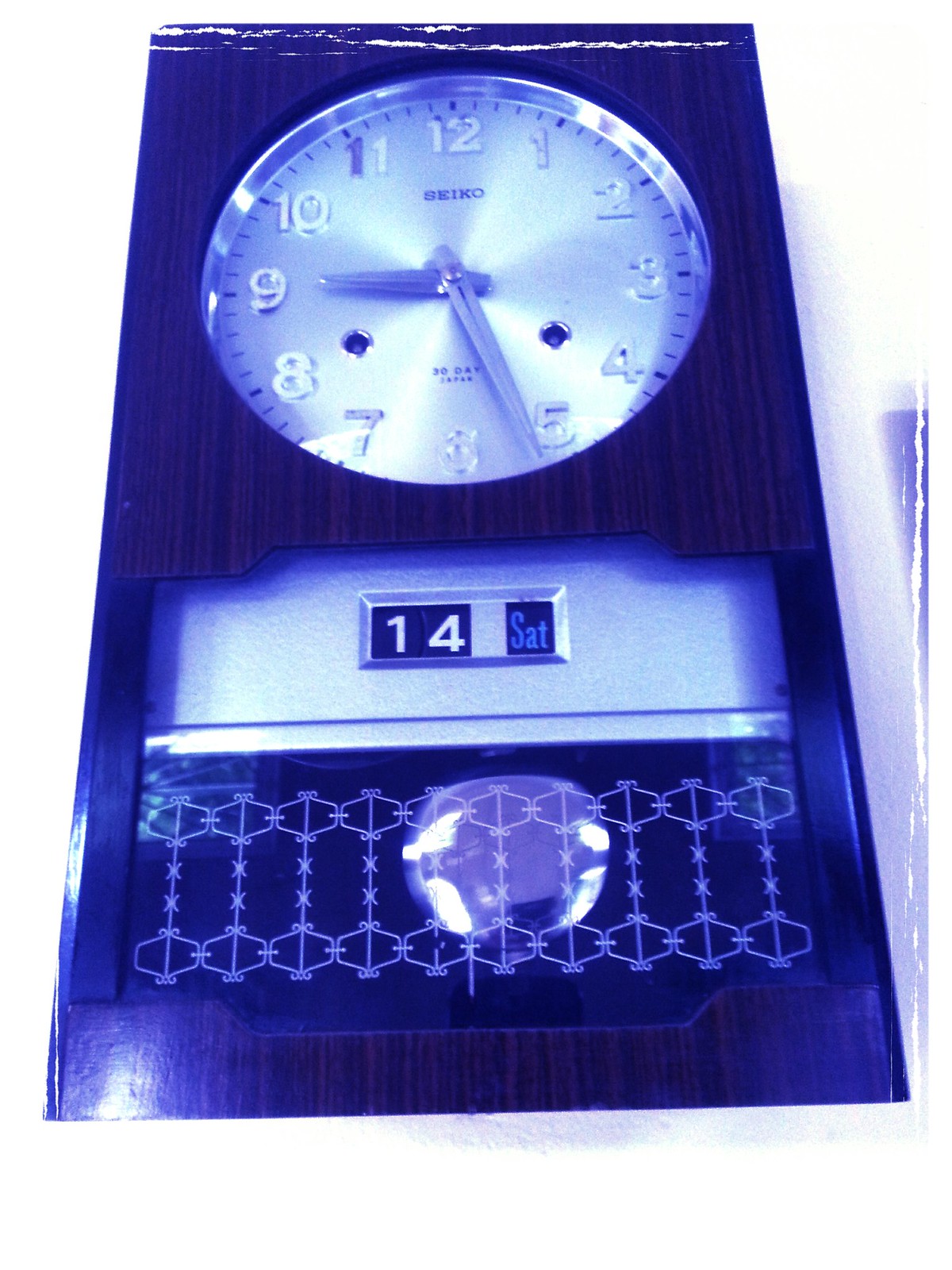This photograph depicts a modern grandfather-style clock with a distinct blue filter that casts a bluish hue over the entire image. The clock is housed in a rectangular wooden frame with ornate etching on its glass front panel. The clock face, positioned in the upper middle section, is circular and has a silver background. It prominently displays the brand name "Seiko" beneath the 12 o'clock mark. The numerals on the clock face are silver, with the number 11 being notably darker than the others. The time displayed is approximately 9:30. Below the clock face, a pendulum can be seen, slightly off to the right, appearing to move. The bottom portion of the clock features a digitized date display indicating "14 Saturday" (S-A-T). Intriguingly, there are keyholes visible for making adjustments. Despite its dimensions and modern styling, the clock evokes the classical form of a grandfather clock.